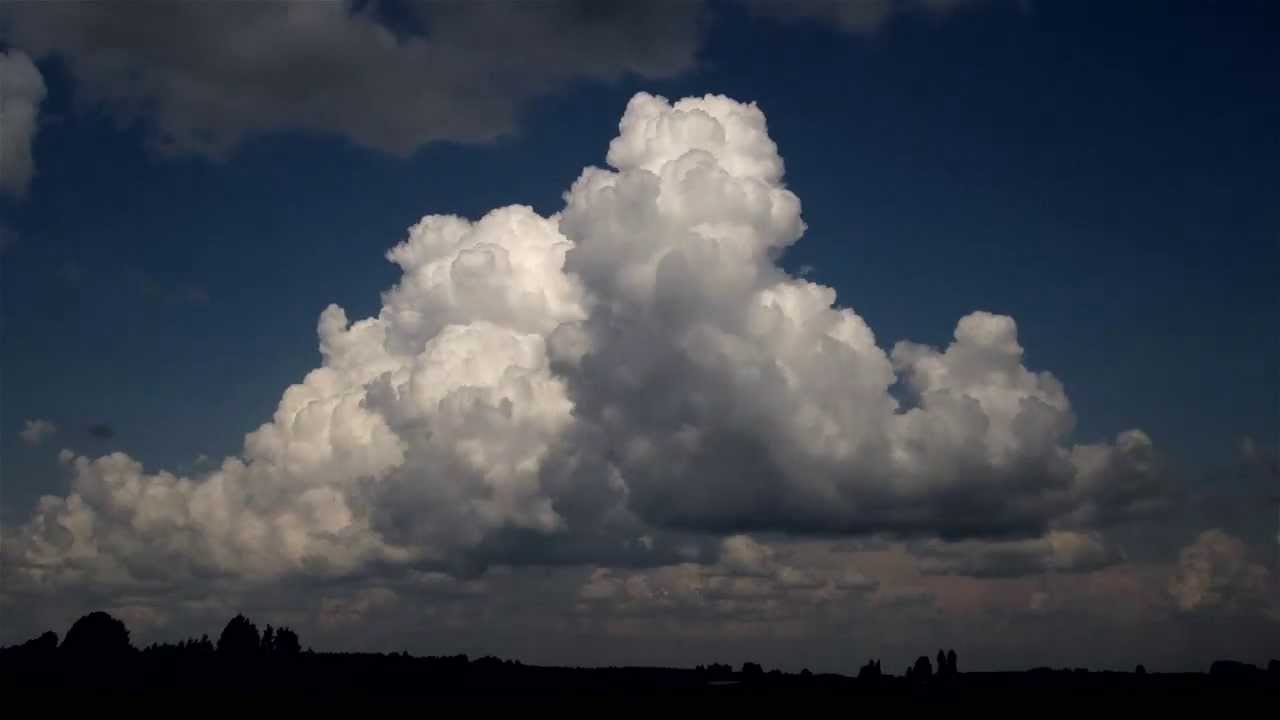The image captures an outdoor scene dominated by a monumental, fluffy, white cloud at the center of a darkening blue sky. The focus is on the enormous cloud, which appears to be lit from within, making it stand out against the darker gray clouds framing the top of the image. Beneath this captivating sky, the landscape is silhouetted in black, with outlines of trees, rocky formations, and possibly a few buildings barely discernible. Despite some pink highlights near the horizon adding a subtle touch of color, the overall palette is limited to varying shades of blue, gray, and white. The scene is devoid of any people or text, leaving the immense cloud as the central figure in a vast, almost otherworldly skyscape.